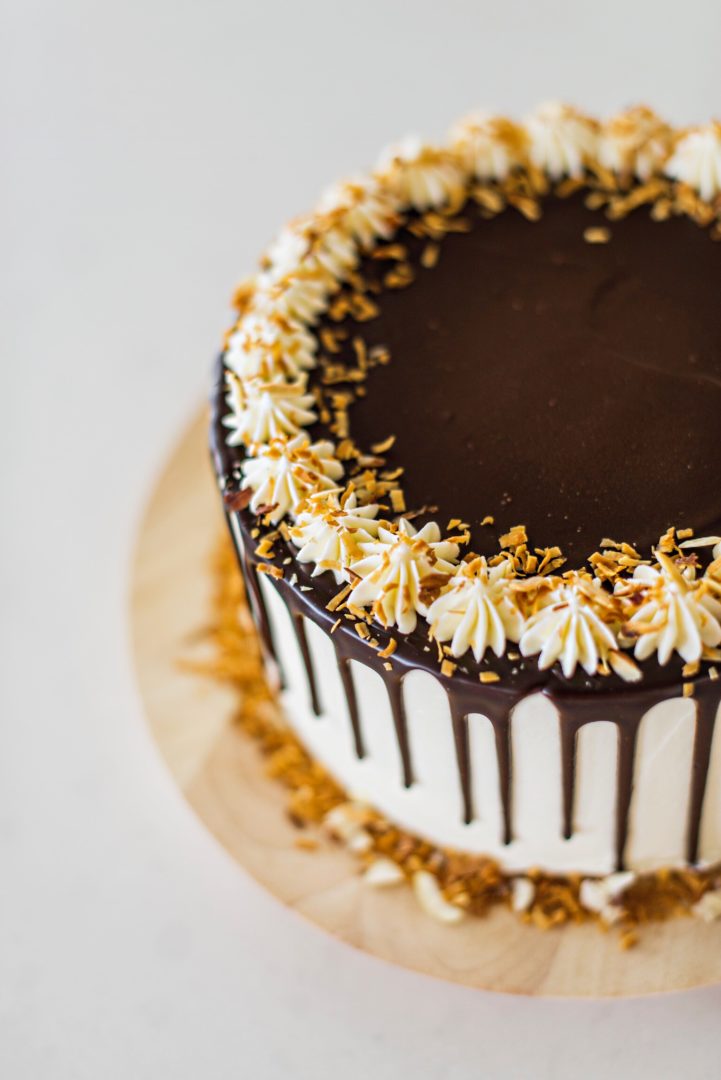This photograph features a close-up of a luxurious, tall, and round cake that dominates the frame with a portion of the right side slightly cut off. The cake rests on a wooden tray against a white background, giving it an elegant presentation. The smooth, white frosting serves as a base layer, while a layer of solidified chocolate has been artfully drizzled over the top, creating visually appealing drip lines down the sides. Around the perimeter of the top, delicate, star-shaped white frosting embellishments encircle the chocolate layer, some of which are garnished with shaved chocolate or coconut. At the bottom edge of the cake, there is a generous sprinkling of toasted nuts, adding texture and a touch of rustic charm. The cake appears fresh, uncut, and about eight to nine inches in diameter, exuding a sense of meticulous attention to detail and craftsmanship.